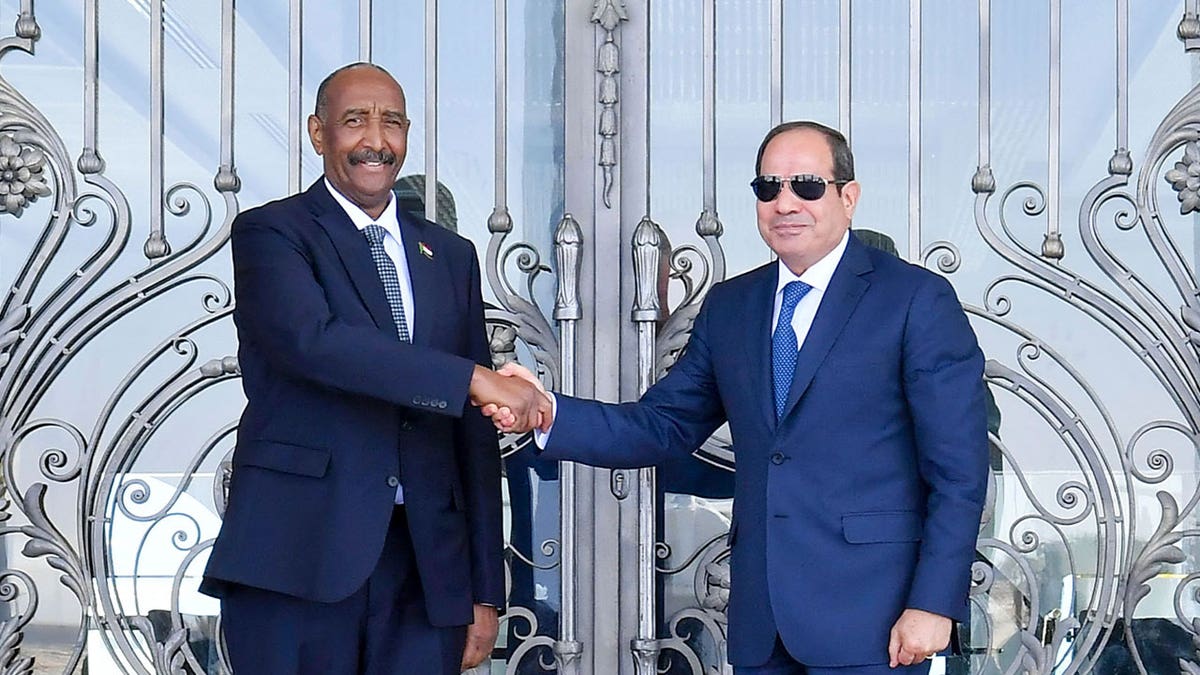This color photograph captures a moment where two men are shaking hands in front of an elaborate silver metal gate made up of intricate glass panels and elaborate filigree. The gate features large, ornate silver handles and a design of straight metal rods that transition into detailed scroll patterns halfway down. The left man, who is black and bald, wears a navy blue suit, a white shirt, and a dark checkered tie with a lapel pin on his left side. The right man, clean-shaven and Caucasian, wears sunglasses, a lighter blue suit, a white shirt, and a lighter blue tie with small white spots. Both men are looking directly at the camera in a portrait-style pose, with their handshake positioned centrally. The silver gate behind them, taller than both men, adds an ornate backdrop to this formal encounter.